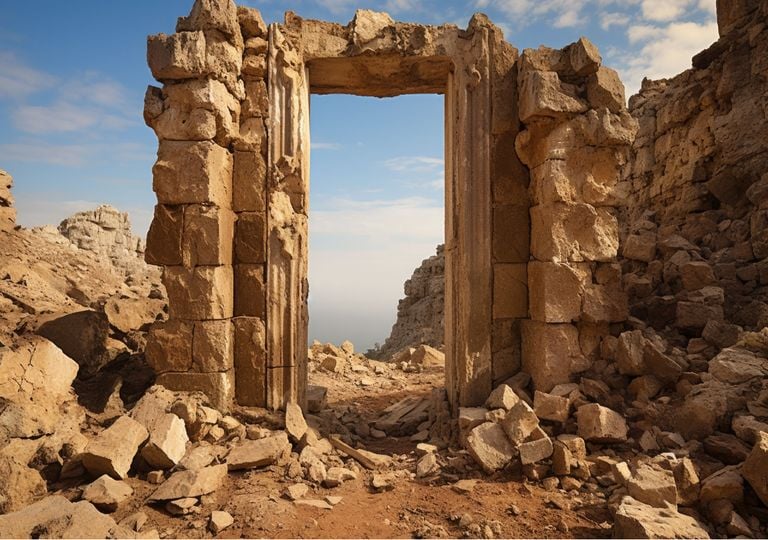This photograph vividly captures an ancient settlement, likely situated in the Middle East, featuring a striking stone doorway made of large, brownish sandstone blocks. The doorway appears as the surviving remnant of a collapsed structure, flanked by walls on both sides. These walls, composed of the same brown sandstone, extend outwards, with an assortment of boulders and broken sandstone blocks scattered across the foreground. The ground itself is covered with reddish-brown dirt, enhancing the earthy tones of the ruins. Dominating the background is a clear blue sky adorned with white clouds, adding a serene contrast to the rugged, archeological landscape. The photograph effectively showcases the remnants of the stone structure amidst a picturesque backdrop, evoking a sense of ancient history frozen in time.